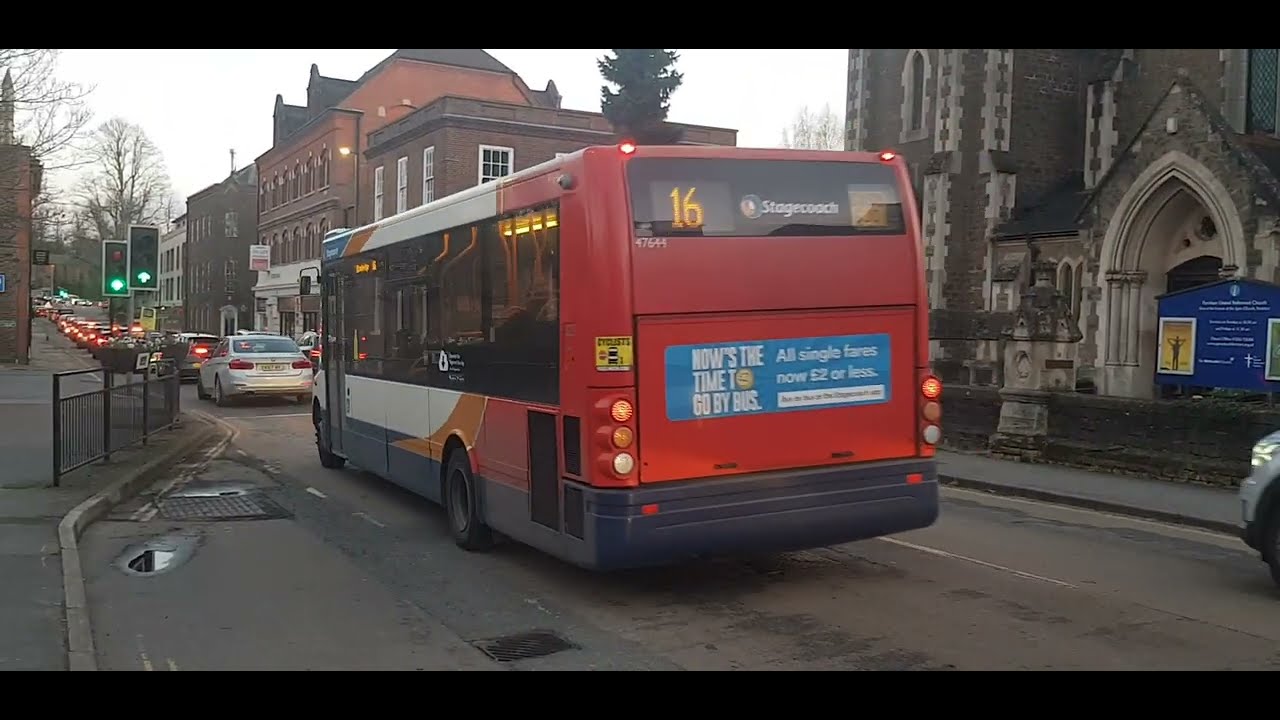In the image, there is a one-way street lined with several stories-high buildings closely packed on each side. Prominently in the foreground is a red bus with stylized dark blue, orange, and white accents, labeled with the number 16 on a digital signage board. The bus is heading away from the viewer, leading a long line of cars with their brake lights on, indicating heavy traffic despite a green light visible from a street sign. Of particular note is an advertisement on the back of the bus stating, “Now’s the time to go by bus, all single fares now two pounds or less,” pointing to a location in England. 

The right side of the street features a significant, old church or cathedral building, suggesting a historical aspect of the city. Meanwhile, on the left, there is black fencing, illuminated street signs with green arrows, and a sidewalk. In the distance, trees devoid of leaves hint at a fall or winter season, further confirmed by the presence of small puddles amidst potholes on the road from recent rain. In the sky, an overcast whiteness encloses the scene, creating a slightly muted atmosphere. The buildings further down the street exhibit varying shades of reddish, brownish, and white, adding to the urban backdrop.